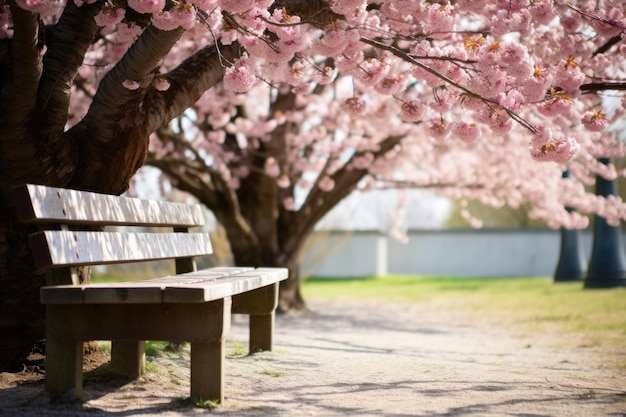In this serene photograph, we observe a well-worn, flat path flanked by an expanse of light green grass. To the left of the path is a wooden park bench with four legs, three wooden slats for the seat, and two slats on the backrest, inviting visitors to rest. The bench is positioned directly under the wide canopy of a stunning tree adorned with pink blossoms, likely cherry blossoms or dogwood flowers. These blooms are fully intact on the branches, creating a lush overhead canopy.

The scene is bathed in muted daylight due to an overcast sky, though ample sunlight filters through, illuminating the bench and the tree's blossoms. Far in the background, a white wall with gray trim is visible, adding a subtle architectural element to the natural setting. To the right of the wall, two large, man-made structures, possibly the base of light posts, stand without their tops visible due to the low-hanging branches of the blossomed tree. Additionally, there are trees with green leaves further in the distance on the right, though they are too far away to identify distinctly. The overall composition captures a tranquil and inviting park scene, perfect for leisurely contemplation.